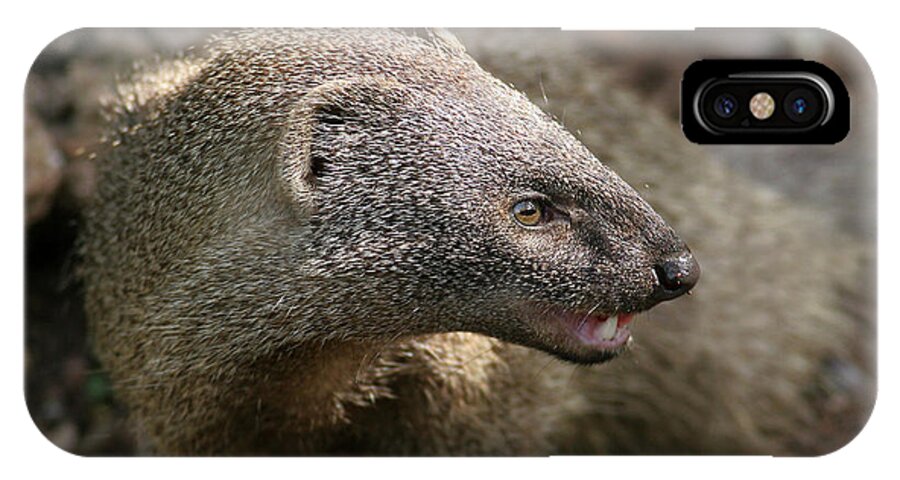The image depicts a rectangular, curved-corner cell phone case featuring a detailed photograph of an animal, resembling a honey badger or otter, with brown, fur-covered body and expressive features. The animal, positioned horizontally with a head turned backward, reveals a side profile. Its mouth, slightly open, exposes a lower fang, and a partially visible eye with a horizontally slanted pupil. The nose is brown, elongating past the mouth. The fur transitions from brown near the body to interspersed gray and black around the face. The small, almost rainbow-shaped ears are tucked close to the head. In the top right corner of the case, there is a cutout for the camera, shaped as a black oval housing three circular, reflective lenses. The detailed craftsmanship makes the creature’s expression appear intense on the case, which measures approximately six inches in width and two to three inches in height.